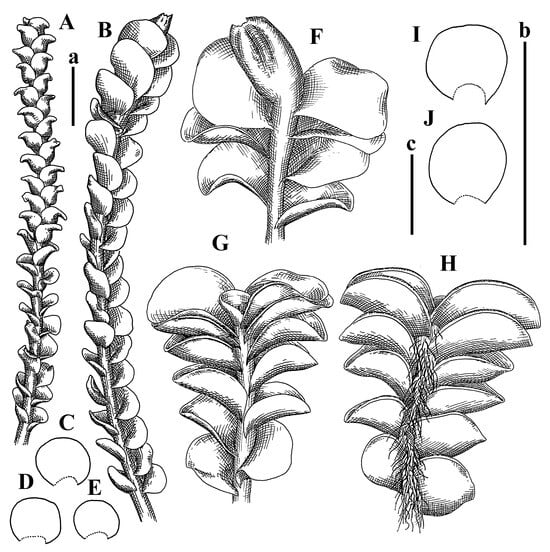The illustration is a detailed black-and-white drawing reminiscent of an image from a science textbook or journal. It consists of a series of labeled pictures depicting different stages of plant growth, organized with capital letters from A to J and lowercase letters a, b, and c. In the top left corner, images labeled A and B feature long stems with leaves growing on each side. Below these, illustrations C, D, and E display almost circular shapes, possibly representing leaves in early development stages. Moving to the center, F and G present a closer view of stems and leaves, which are more developed and similar to the ones shown in A and B. The lower right corner houses image H, similar to G but with small hairy projections. The top right corner contains images I and J, larger circular representations akin to C, D, and E, but in greater detail. The entire drawing is meticulously labeled and depicted in shades of black and gray against a white background.